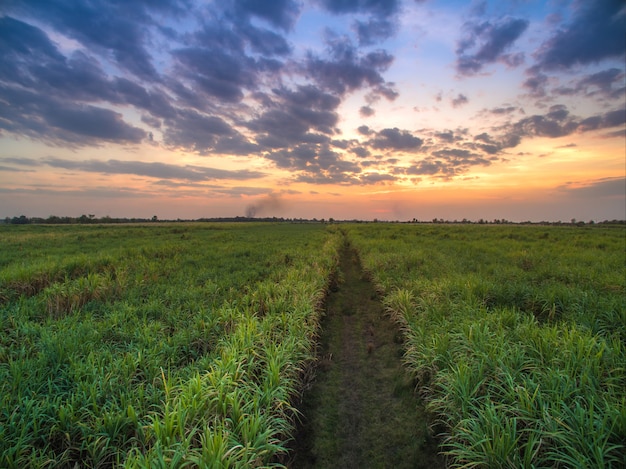This landscape photograph, taken in the countryside during a stunning sunrise or sunset, showcases a picturesque field that appears to be used for farming. The lower half of the image is dominated by lush green plants organized in rows, divided by a central path of trampled grass or dirt that leads the eye towards the horizon. The upper half features an expansive sky painted in vibrant shades of purple, blue, pink, yellow, and orange, hinting at the time of day. Scattered, fast-moving clouds with interesting swirls add a dynamic element to the scene. In the far distance, the silhouetted outline of tiny trees is visible, and a thin trail of smoke rises from an unknown source, adding a subtle touch of mystery to the tranquil ambiance. The contrast between the rich green crops and the colorful sky creates a visually striking and serene image.